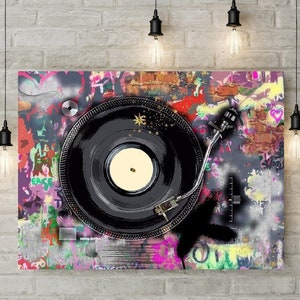The photograph captures a striking piece of wall art mounted on a light, whitish-grey painted brick wall, illuminated by four bright white bulbs in black sconces. The artwork creatively portrays an old-fashioned turntable with a black record spinning under the needle, depicted as if the viewer is looking straight down onto the turntable. The piece melds realistic elements with graffiti-style, abstract expressions in vibrant blues, greys, reds, and yellows, creating a captivating pop art effect. The turntable's white interior contrasts sharply with the colorful, expressive background, making it the focal point of this modern, indoor studio setup.